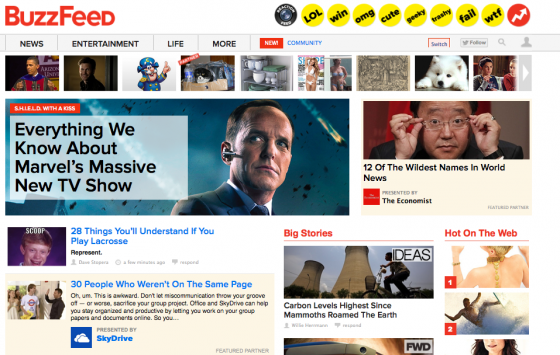The screenshot captures the homepage of BuzzFeed, prominently featuring the BuzzFeed logo in red. Surrounding the logo are 10 circles, sequentially: the first circle is black, followed by eight yellow circles with black writing, and the final circle is red with a white arrow inside.

At the top of the page, there is a search bar with categories including "News," "Entertainment," "Life," and "War." Below the search bar, a series of news articles are displayed, with headlines such as "Everything We Know About Marvels and SNTV," "12 of the Wildest Names," "Hanukkah," "Web," "Big Stories," "28 Things You'll Understand If You Play Lacrosse," and "30 People Who Aren't on the Same Page."

The articles are grouped into sections; one particular section is highlighted in blue with accompanying images. The section prominently features red text headings such as "Big Stories" and "Hanukkah Web." The entire interface is vividly colored, with each article presented within its own distinct color tone. Additionally, at the top of the page, there are about 12 clickable photo links.